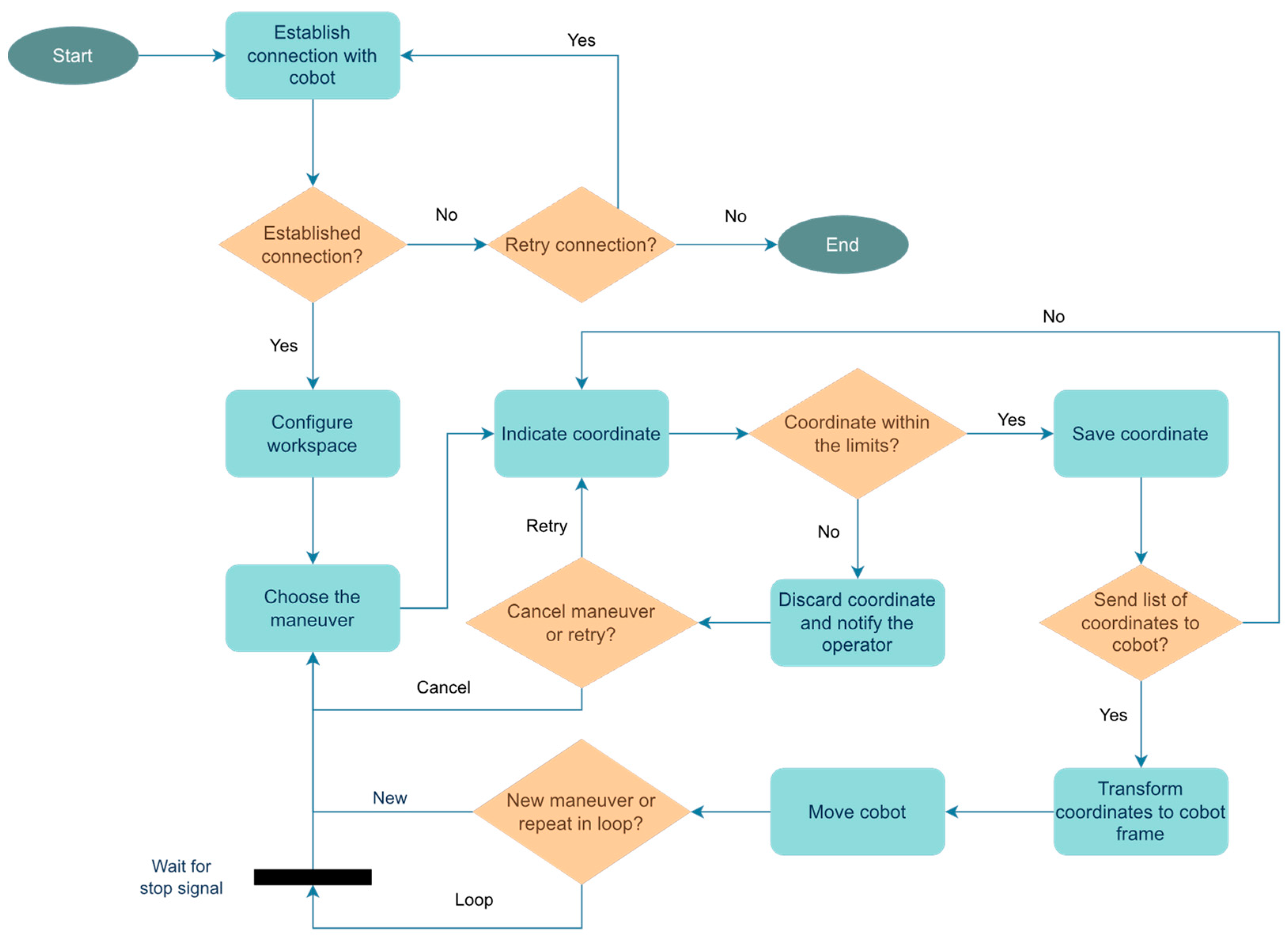This detailed decision chart, suitable for a slide presentation or textbook, serves as a flow diagram for establishing a connection with a Cobot. Starting at the upper left corner, an oval labeled "Start" initiates the process. The chart utilizes a combination of blue arrows to guide through various steps, light-blue rectangles, and orange diamonds, each representing different decision points or actions.

The flowchart is organized into five rows, each containing approximately four decision points. The initial step is establishing a connection with the Cobot, as indicated in a rectangular box. If the connection fails, the chart directs to a diamond shape prompting retries until a successful connection is established. 

Upon a successful connection, subsequent steps include configuring the workspace, choosing a maneuver, and indicating coordinates. The flow diverges based on the coordinate's acceptability: if within limits, coordinates are saved and sent to the Cobot; if not, they are discarded, and the operator is notified. 

The process continues, enabling transformations, movement, and retries as necessary. If new maneuvers arise or a loop is established, it allows for repetitions or cancellations. At the very end, the flowchart culminates at a black bar in the bottom left corner indicating to "Wait for stop signal."

The primary colors—dark teal for the oval start, light blue for rectangles, and peach for diamonds—aid in visually distinguishing the chart’s elements. The detailed structure balances comprehensive guidance with pathways for retries, notifications, and operational commands, creating a robust roadmap for managing the Cobot connection process.